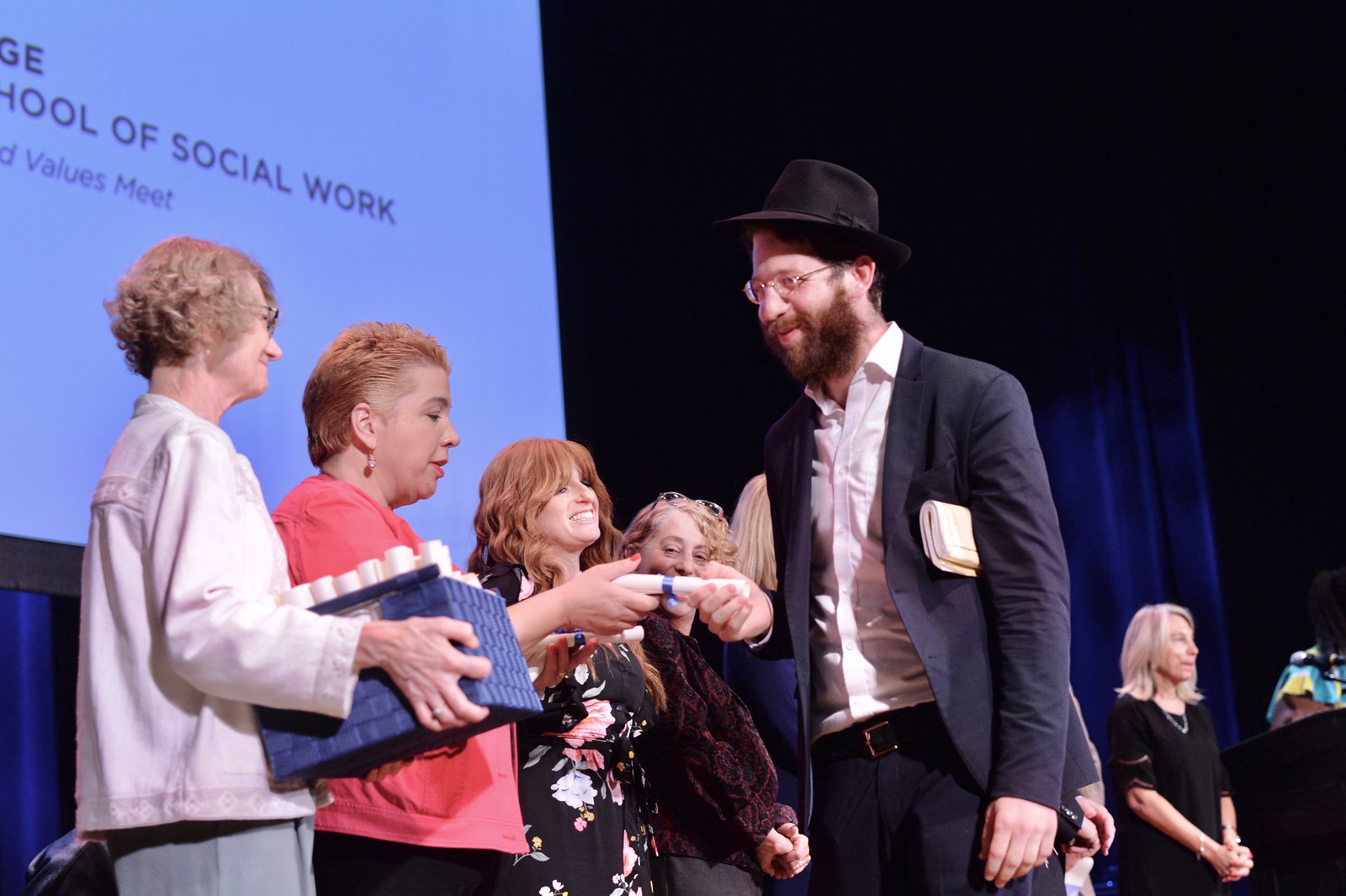On a blue-curtained stage, a graduation ceremony is taking place. A bearded man in a blue blazer, white shirt, and dark pants is receiving a rolled-up document tied with a blue ribbon from a woman next to another woman holding a container full of similar documents. He has a white booklet tucked under his left arm and is wearing a black trilby hat and glasses. Six women, likely administrators or teachers, stand in a row, participating in the ceremony. A partially visible projected screen in the background reads "School of Social Work and Values Meet," suggesting that the event celebrates graduates from a social work program.